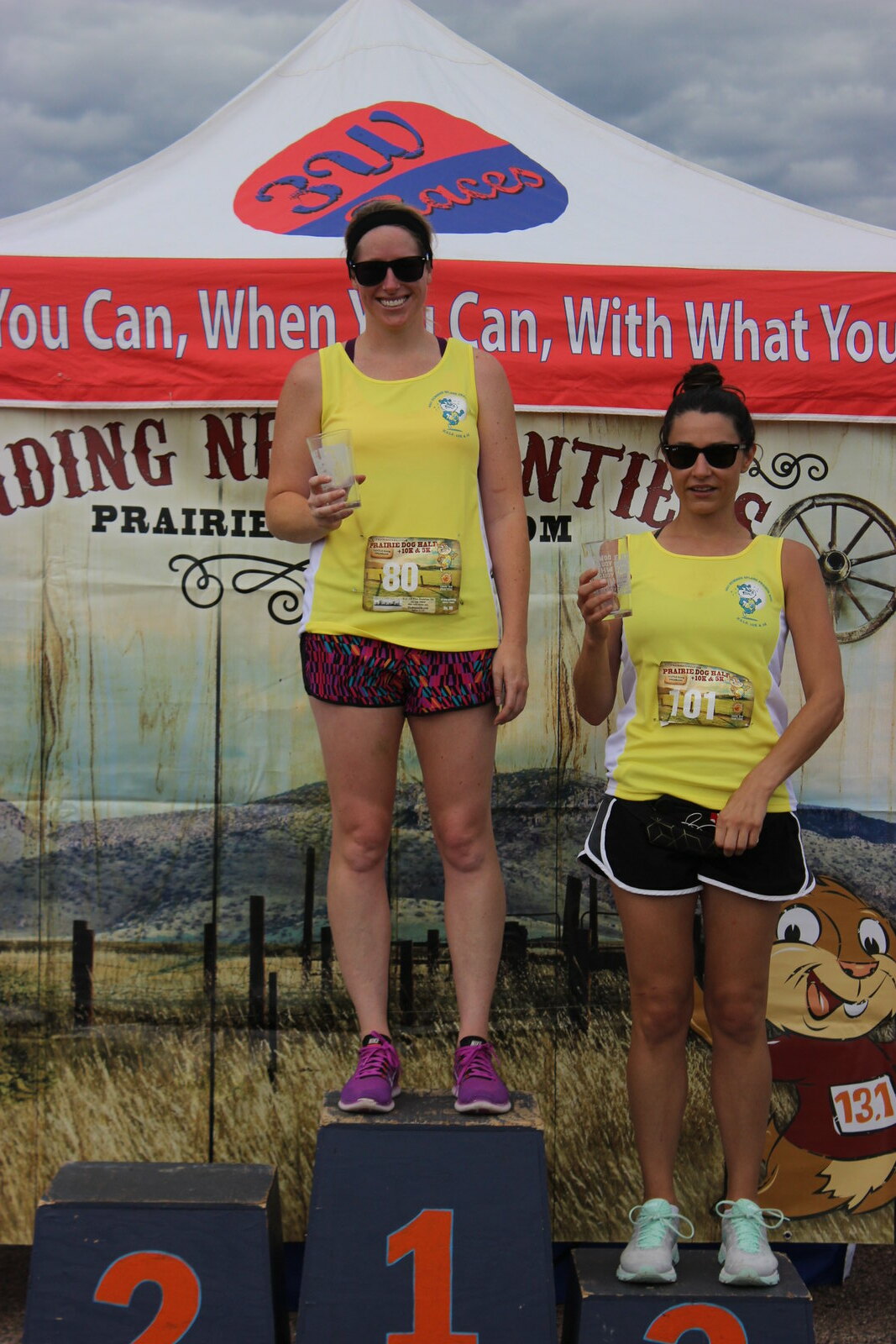In this color photograph taken outdoors under a cloudy sky, two women are standing proudly on a three-level podium in front of a white pop-up tent adorned with various banners and advertisements. The tent features a distinct 3W Races logo on its white top, with a red banner along the edge reading “You can, when you can, with what you” in white text, though partially obscured by the women. Below this banner, in an old western font, the word "frontier" can be made out, along with a mural depicting a prairie scene and a numbered cartoon prairie dog.

The women are dressed in coordinated athletic attire, both wearing yellow tank tops with race numbers on their bibs. The woman on the left, standing on the first-place podium (number 1), wears bib number 80 and smiles brightly at the camera. She has light-colored hair pulled back by a black band and sports multicolored running shoes and shorts. The woman on the right, occupying the third-place podium (number 3), has her hair styled in a high messy bun and is dressed in black running shorts with white accents and mint-green laced shoes. She wears bib number 101.

Both women are accessorized with dark sunglasses and are holding clear glasses of water in their right hands. There is no one on the second-place podium (number 2). The setting suggests they have just finished a race, likely a 10K or 5K event, as hinted by the details on their bibs and the awards they're holding.